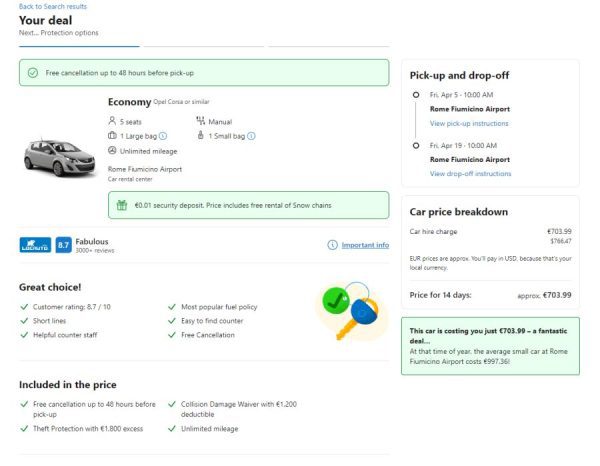This image displays a detailed page featuring comprehensive information about a vehicle rental. Central to the image is a review and specification section that highlights various aspects of the vehicle and rental terms. The page includes texts and labels such as "Back to search results," "Your deal," and emphasizes the convenience of "Free cancellation up to 48 hours before pickup."

Key details of the vehicle are presented, such as its class (economy), seating capacity (5 seats), and baggage allowances (1 large bag, 1 small bag). The rental offers unlimited mileage and features a manual transmission. The financial specifics mention a minimal security deposit of 0.01 euros and include free rental of snow chains in the price.

The vehicular rating stands at 8.7, described as "fabulous" and based on over 3,000 reviews. Further ratings emphasize the vehicle as a "Great choice," with a customer satisfaction score of 8.7 out of 10. Highlights of the rental experience include "Most popular fuel policy," short waiting lines, helpful counter staff, and an easy-to-find counter, all contributing to an overall high level of customer satisfaction.